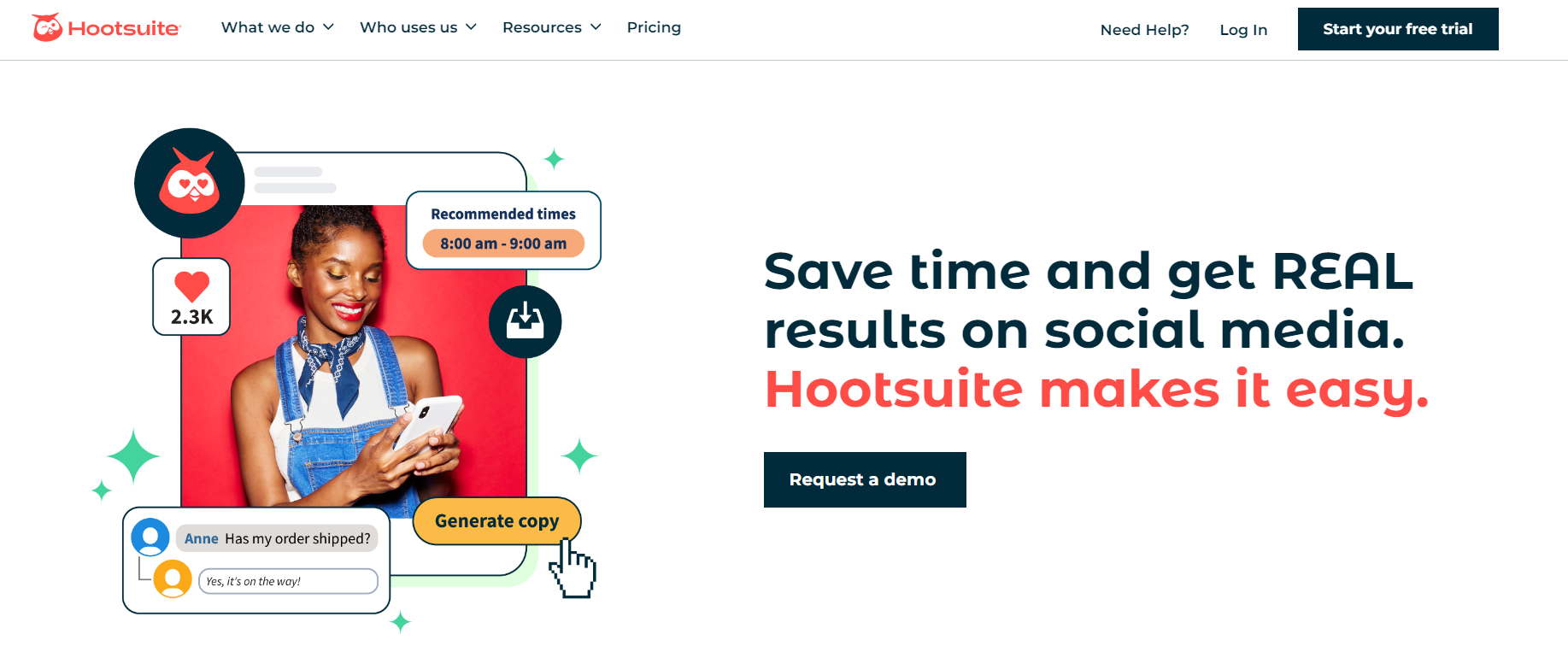This is a left-to-right horizontal image, presumably from a website that can be accessed via a computer or smart device. The background is predominantly white, borrowing the blank canvas from the user's computer screen.

In the upper left-hand corner, the HootSuite logo featuring a red owl icon is prominently displayed. To the right of the logo, navigation links read "What We Do," "Who Uses Us," "Resources," and "Pricing," all in black text. Further to the right, there are additional links saying "Need Help," "Log In," and a black box labeled "Start Your Free Trial."

Back to the left side, there is an image of an African-American woman looking at her phone. The phone screen displays various social media metrics, such as recommended times to post and the number of 'hearts' or likes a post has received. Additionally, a chat interface shows a conversation where a person named Ann asks, "Has my order shipped?" and the response states, "It's on the way," offering a preview of HootSuite's functionalities.

On the right side of the image, bold black text emphatically states, "Save Time and Get REAL Results on Social Media," with "REAL" in all caps for emphasis. Below this slogan, in red text, it says, "HootSuite makes it easy." Finally, at the bottom lies a black rectangular box with white text that reads, "Request a Demo."